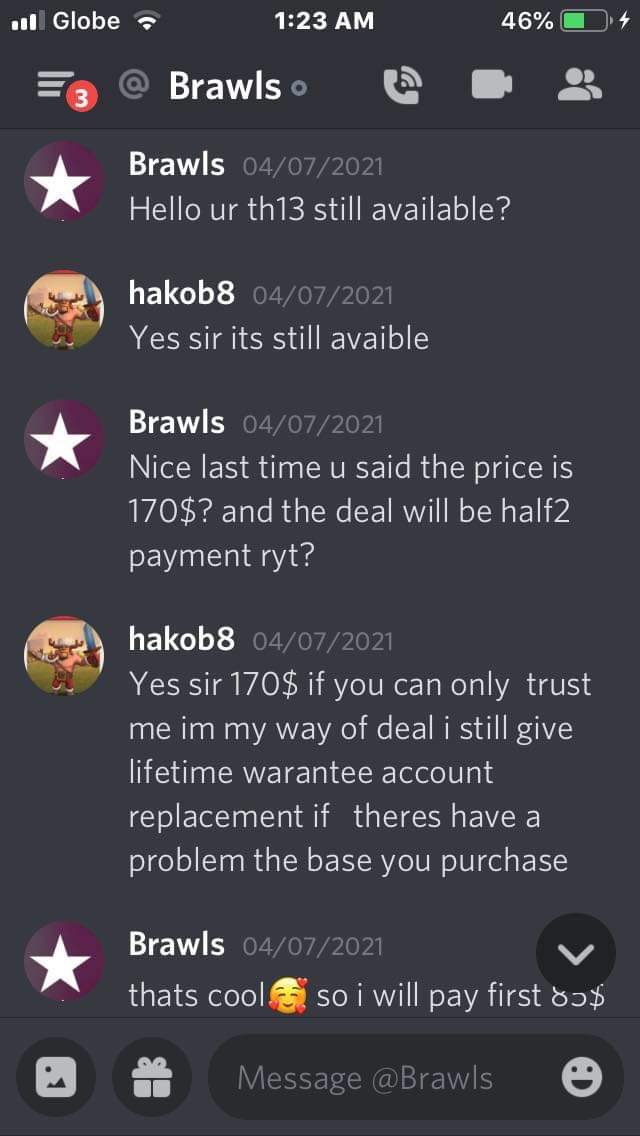In this image, we see a screenshot of an iPhone displaying an active text conversation between two users, Brawls and HackCode8, dated April 7, 2021, at 1:23 a.m. Brawls initiates the conversation by inquiring if HackCode8's TH-13 product is still available, to which HackCode8 confirms affirmatively. Discussing the price and payment terms, Brawls recalls the previously mentioned price of $170, structured into two payments. HackCode8 reassures Brawls of the $170 price and mentions offering a lifetime warranty with account replacement should there be any issues with the purchased base. Brawls agrees to the terms, indicating a payment of the first half, approximately $85, and plans to complete the remaining payment later. The dialogue is displayed with clear timestamps and user identifiers, highlighting the negotiation and agreement process.